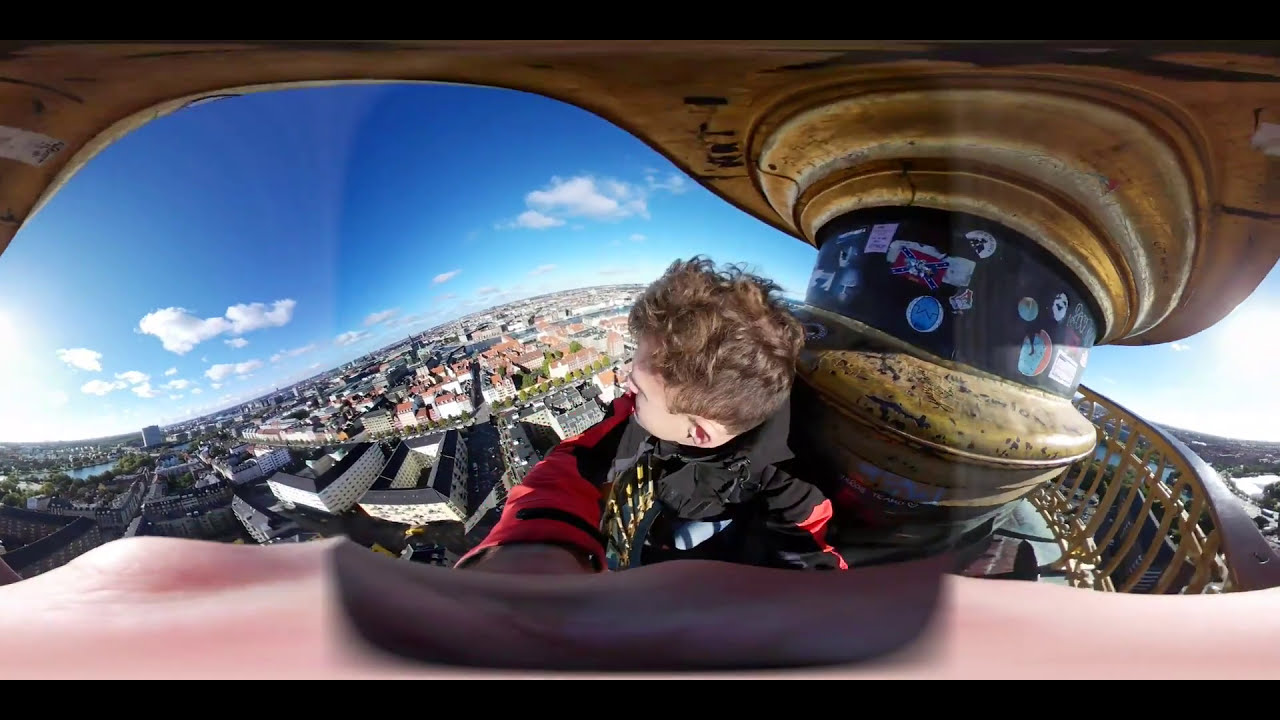In this panoramic image, a somewhat young man with messy brown hair is captured on a high observation balcony overlooking a vast urban cityscape. The man, clad in a red and black coat, is leaning against a worn, goldish-brown post adorned with various stickers and bits of graffiti. He gazes down and slightly to the left, taking in the seemingly endless expanse of buildings and homes below, with streets carefully laid out in a perpendicular grid pattern. The balcony, outlined by a fence, curves behind him, adding depth to the scene. The day is clear with a beautiful blue sky dotted with a few white clouds, enhancing the striking view of the city's brick-red rooftops and detailed structures stretching out to the horizon.